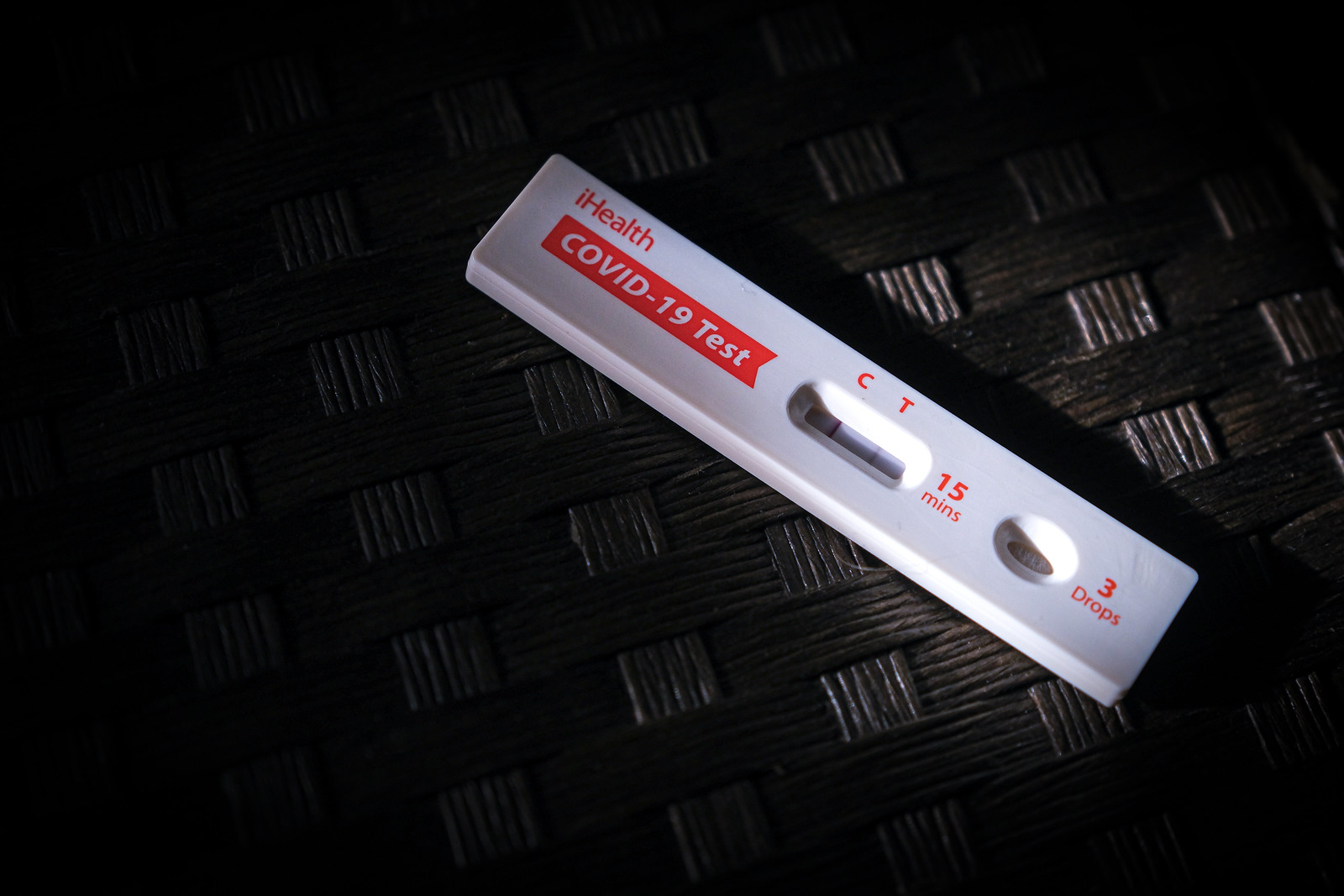The image showcases a COVID-19 test kit placed atop a surface with a basket weave texture. The test kit, predominantly red and white, measures approximately four and a half inches in length. On the left side, the label "Eye Health" is displayed in red, just above a red box containing the text "COVID-19 Test." On the right side of the kit, the letters "C" and "T" are visible, along with a marking that reads "15 minutes." Adjacent to these markings, there is a small well designed to receive a sample, indicating that three drops are required to determine the test's result. This focal point of the image is the COVID-19 test kit itself, with no other objects present in the frame.